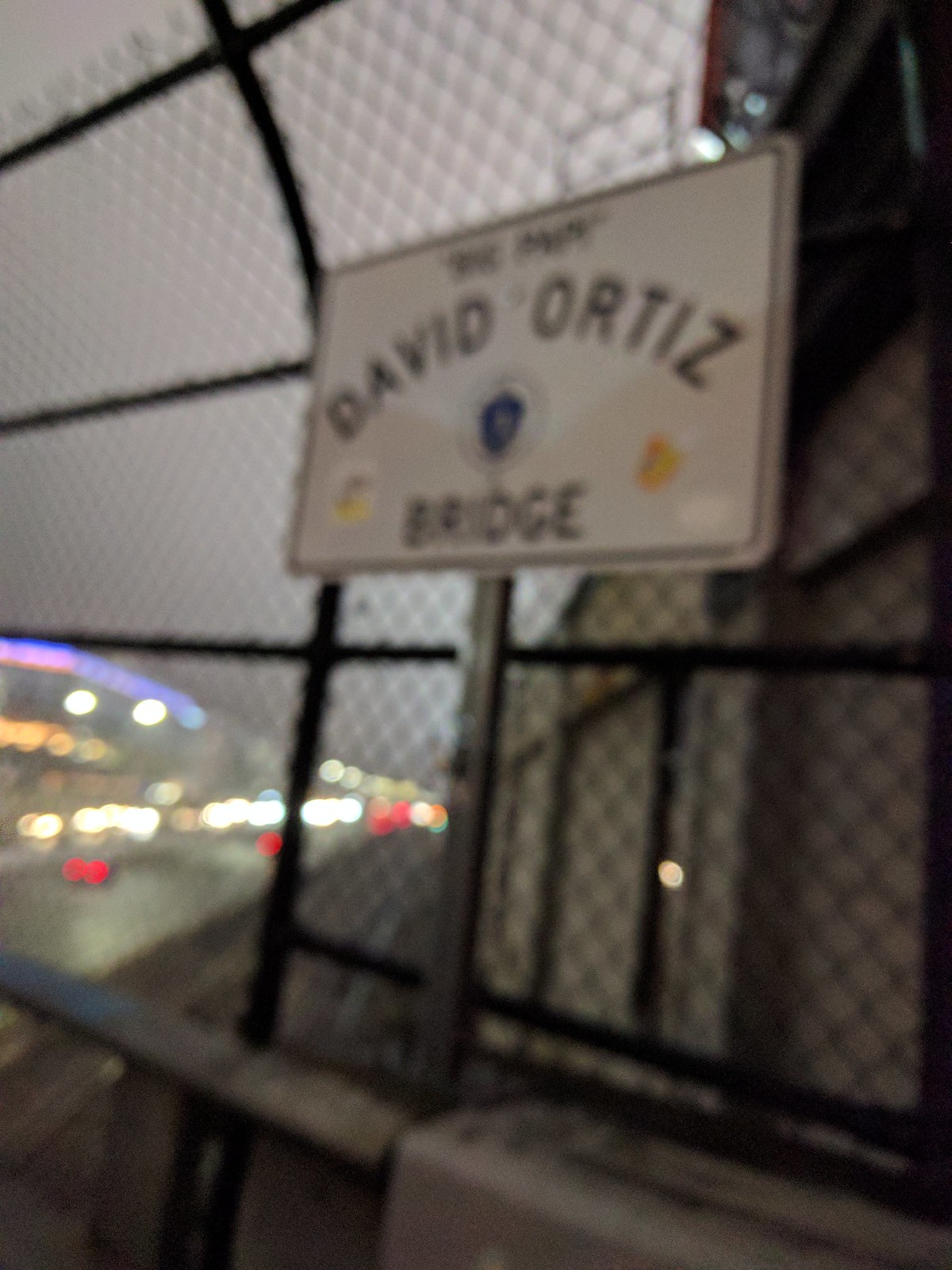The image captures a sign on a gated bridge named the David Ortiz Bridge. The bridge is closed off by a black fence that extends across its entirety. The white sign prominently features the name "David Ortiz" along with an insignia in the center, marked by blue and yellow details, and the word "Bridge" at the bottom. The foreground is somewhat blurred, possibly due to poor camera settings or an overcast, rainy day. In the background on the left, blurred headlights and taillights of multiple cars indicate traffic moving on adjacent streets. The blurred effect contributes to a sense of motion and a dreary atmosphere.